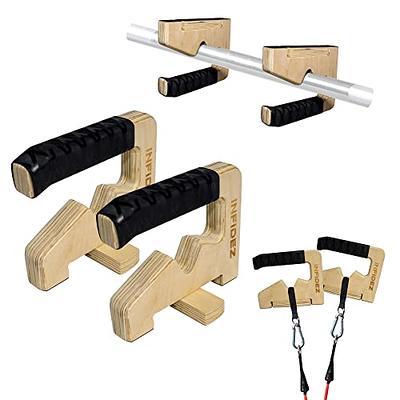The image features small wooden hangers, with the lower left corner providing a close-up view of two of the items. The right Side of each hanger is engraved with the word 'Inpedez,' spelled I-N-P-I-D-E-Z. Each hanger has a distinctive design: one end boasts a long black handle, while the other end features a wooden handle with a carved notch. In the far right corner of the picture, two hangers are shown side by side, hanging on a closet bar with their black handles extending underneath. The lower right section displays the hangers flipped over, revealing thin black straps dangling in the center cutout area of the hanger, showcasing their versatility.